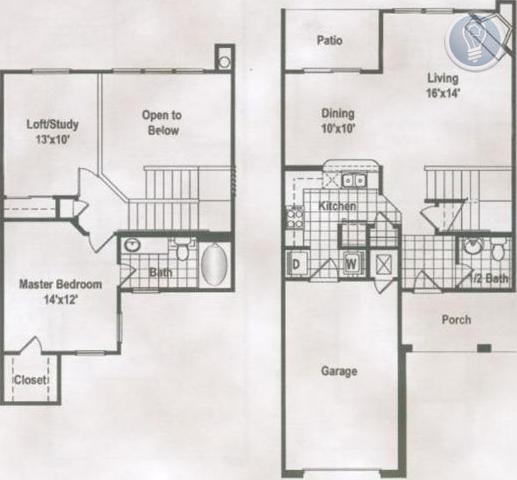This architectural drawing depicts a detailed layout of a two-story home, presented in black lines of varying thickness on a white background. The image provides a clear view of both the lower and upper stories, with the lower floor plan displayed on the right and the upper floor plan on the left.

In the lower floor plan, a prominent garage space occupies the front left portion of the building. Adjacent to the right of the garage is a smaller porch area. The garage provides access to the interior of the home through two doors, one leading directly into a small closet-like area and the other into the main living spaces. Additionally, the porch also features a door connecting it to the home's interior.

Inside, the garage opens up into the kitchen area. Above the kitchen is a 10 by 10 dining area, which seamlessly transitions into a larger, open-plan 16 by 14 living room situated to the right of the dining area. The living room, extending more spaciously than the dining area, also includes a horizontally rectangular patio situated above the dining area and to the left of part of the living room.

The upper story consists of three full rooms and additional features. A master bedroom measuring 14 by 12 sits alongside a 13 by 10 loft study. A smaller bathroom is also included, though not as extensive as the other rooms. There is a large open space on the right side of the upper floor, which includes the outline of a staircase. This design allows for an overlooking view from the second floor onto the open living room below, providing a cohesive and open ambiance throughout the home.